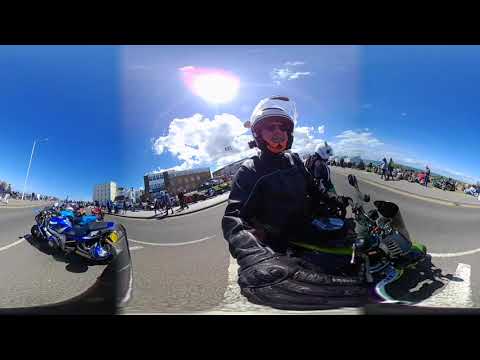In the photograph, a man sits on a motorcycle, centrally positioned on a dark black asphalt road marked with white lines. He's clad in a black leather jacket, black gloves, and a white helmet with a clear visor raised up, revealing his sunglasses and mustache. A microphone is attached to his helmet. In the left background, a blue and white touring motorcycle is parked. The scene appears to be a gathering of bikers, as many people can be seen milling around in the background, some near buildings in the distance. Above, a bright blue sky with scattered white clouds dominates the top of the frame, with the sun shining through slightly blurred, creating a shaft of light down the center of the photo.